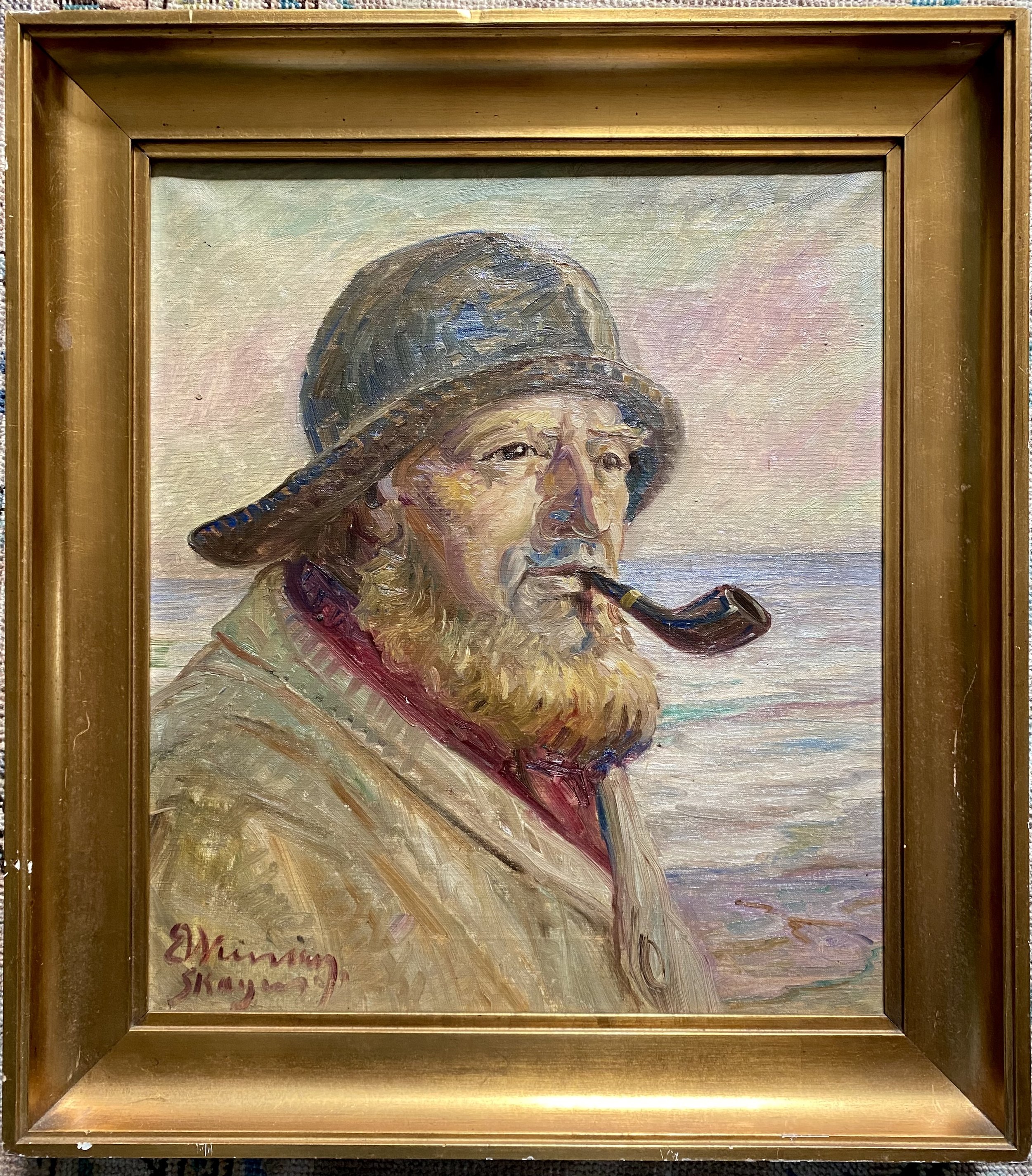This photograph showcases a painting of an older man with distinct nautical characteristics. The painting is framed in a simple, thick gold frame that shows signs of wear with scratches and chips. The canvas is slightly taller than it is wide and does not appear to be protected by glass. The subject of the painting is a man who seems to be a sailor or a man of the sea. He sports a long, bushy blonde beard, complemented by bushy golden eyebrows and a subtle mustache. He wears a dark, floppy bow hat with the brim facing backward. His attire includes a light yellow-brown coat covering a red shirt. In his mouth is a black smoking pipe adorned with a gold strip. The man is posed gazing to the side, revealing a profile view to the audience. The background of the painting features a serene ocean scene with crashing waves and a sky tinged with hues of whitish-green and red. Additionally, there is a signature at the bottom right of the painting, though it is illegible. The combination of the man’s attire and the marine background firmly situates the subject in a maritime context.